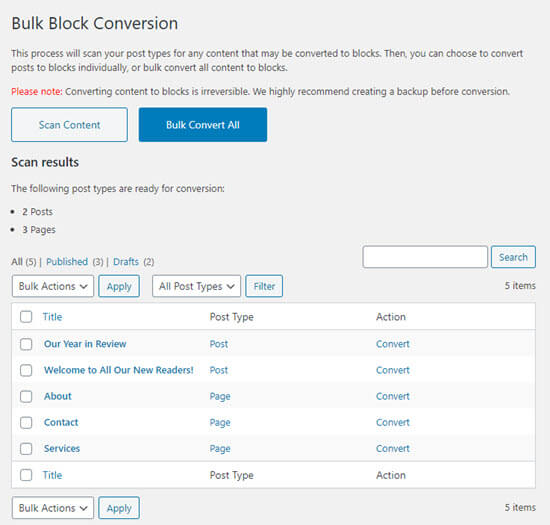**Image Description: WordPress Bulk Block Conversion Interface**

The image is a large square with a gray background, depicting the interface for bulk block conversion in WordPress. 

At the very top, a heading reads "Bulk Block Conversion" in bold text. Below the heading, an informational message explains, "This process will scan your post types for any content that may be converted to blocks. Then you can choose to convert posts to blocks individually or bulk convert all content to blocks." 

Highlighted in red, another warning states, "Please note converting content to blocks is irreversible. We highly recommend creating a backup before conversion."

Two main action buttons are displayed beneath the warning. A gray button labeled "Scan Content" and a blue button labeled "Bulk Convert All." 

Following the buttons, a section titled "Scan Results" lists the content ready for conversion: "The following post types are ready for conversion: 2 posts and 3 pages." 

At the bottom, there is a white rectangle containing a list of the posts and pages to be converted. The first post is titled "Our Year in Review" and the second post is "Welcome to All Our New Readers." The three pages listed are: "About," "Contact," and "Services." 

It appears the user is in the process of choosing to bulk convert these posts and pages, as indicated by their selection of the "Apply" and "Filter" buttons.